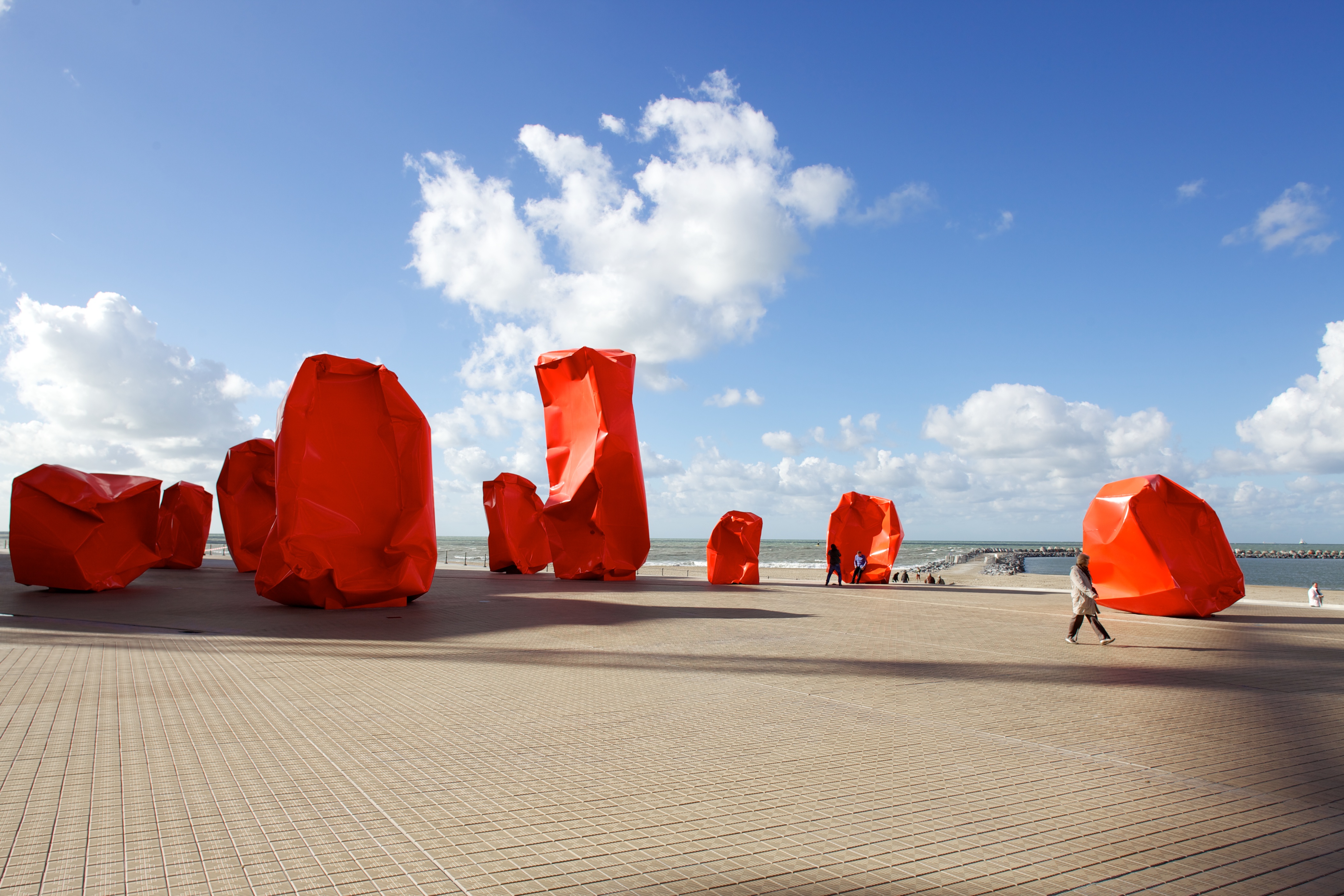The image captures a vibrant art installation set against the backdrop of a serene beach and boat harbor. The sculptures, resembling crumpled paper and bright in a striking shade of red or orange, are constructed from material that could be either plastic or metal. They vary in size and shape, with some appearing as balled-up wads, and others as long rectangular forms. One prominent piece in the center features a concave section where a person is seated. Another towering structure in the middle stands twice as tall as the people around it. A woman in a tan overcoat and white walking shoes is seen strolling past the sculptures. The installation is arranged on a spacious, teal-tiled patio with most pieces gathered on the left side of the scene. The background showcases a picturesque view of the ocean, a jetty marking the harbor, and a beautiful sky adorned with clouds, adding to the overall ambiance.